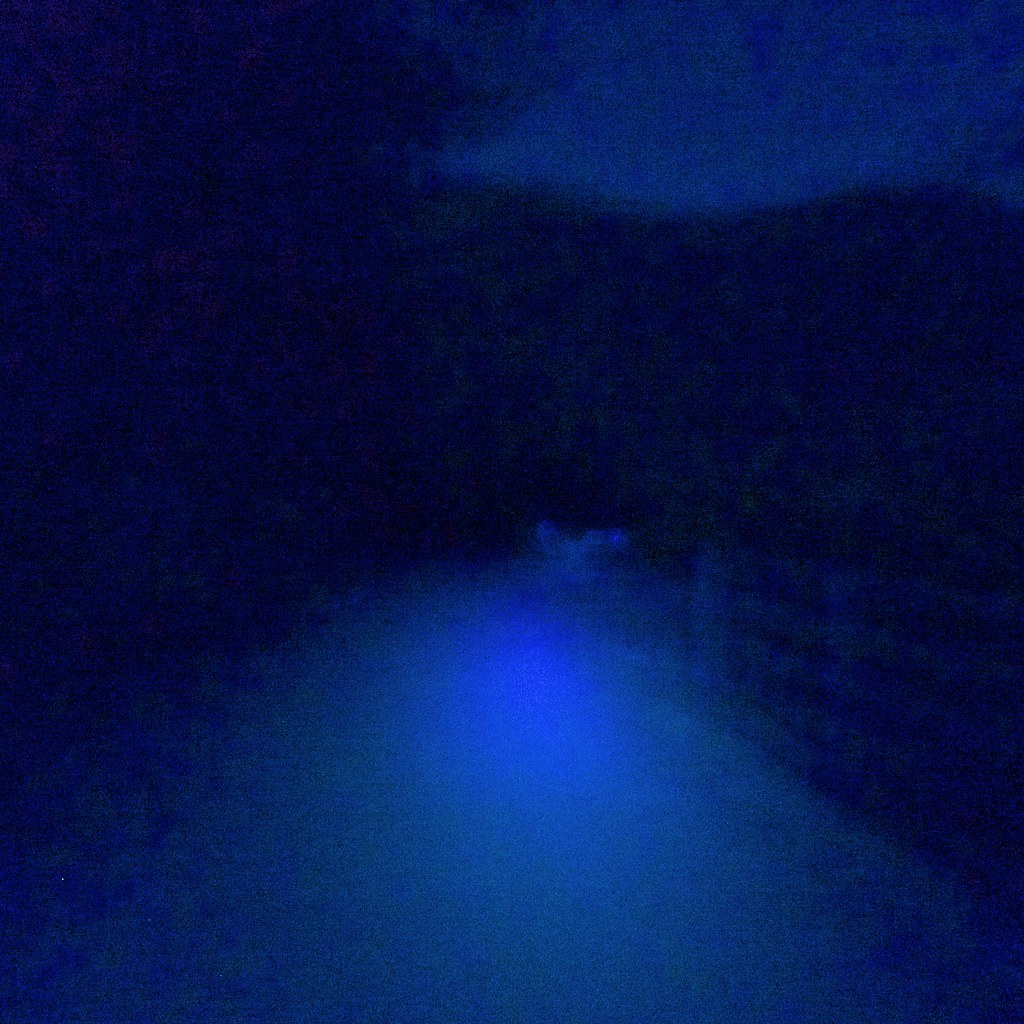The image showcases a square canvas predominantly filled with deep navy hues, creating a moody and introspective atmosphere. In the lower third, just slightly above the bottom edge, a vibrant, brighter puff of blue emanates subtly downward and slightly upward, introducing a gentle luminosity to the otherwise dark composition. This puff of blue gives the appearance of an ethereal light source pushing through the darkness. Towards the top right corner of the canvas, the navy backdrop gradually transitions into lighter blue tones, reminiscent of a distant horizon merging into a twilight sky. The interplay between the dark and light blues across different sections of the canvas suggests a delicate balance between obscurity and clarity, evoking a sense of depth and infinite space.